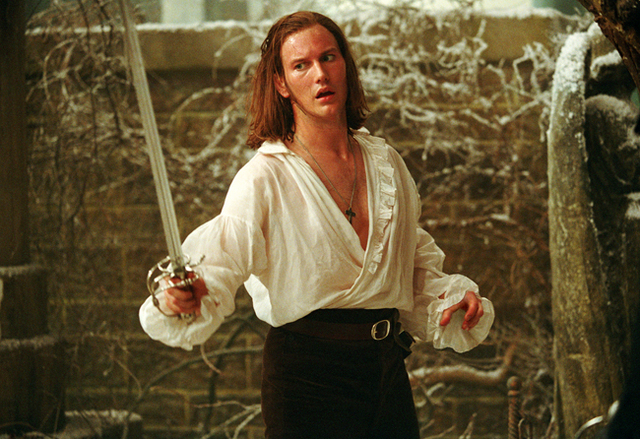In this color photograph, a man stands dramatically before a low stone wall covered in vines and dead branches. Dressed in tight black pants with a silver-buckled black leather belt, he wears a frilly white blouse open at the chest, revealing a gray necklace that ends in a black cross. His long brown hair frames his intense expression as he wields a silver sword prominently in his right hand, while his left hand is raised to his belt level. The background is characterized by a brick wall that rises to his height, topped with stone and dusted with frosty vines. On the right side of the image, the frosty wings of a partially visible statue peek through, while a rounded stone support pillar adds balance to the left side of the scene. The detailed textures and composition create a striking, almost medieval atmosphere.